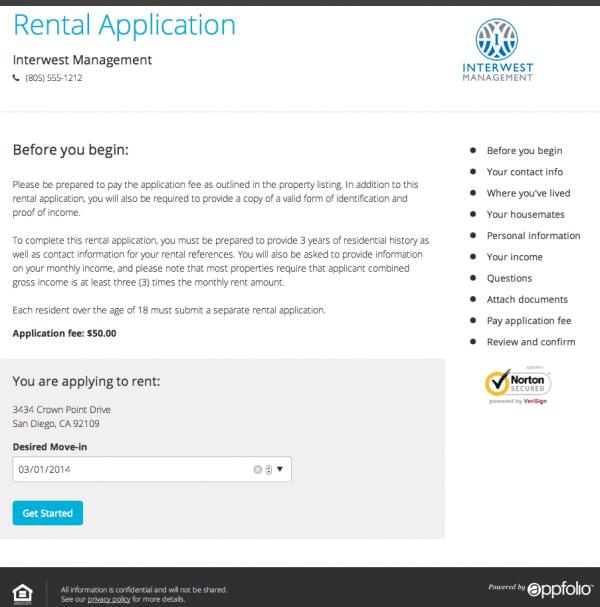This is a detailed screenshot of a rental application form for Enter West Management. At the top, a solid black line separates the header from the application. Directly below, the text "Rental Application" appears in turquoise blue, followed by "Enter West Management" and a contact phone number accompanied by a telephone icon. On the right side, a logo displays "Enter West" in blue lettering with a blue and gray sign, underneath which the word "Management" is written.

A thin, light gray line demarcates sections of the page. Below, there is a heading in black text saying "Before You Begin," followed by a detailed description of preliminary steps. Further down, the application fee is stated in bold black text as "$50," followed by a light gray box indicating the statement: "You are applying to rent." The specific rental address is shown in light gray, alongside a bold, black start move-in date of "3-1-2014." An arrow icon directs attention downward.

A prominent blue box with white text invites the user to "Get Started." At the bottom, a black bar contains icons and links related to terms and policies, as well as the website, demarcated by a house icon.

The right side features a checklist titled "Before You Begin," which enumerates necessary information categories: your contact info, previous residences, housemates, personal information, and income questions. Many descriptors trail off incompletely, suggesting some missing data or incomplete form fields.